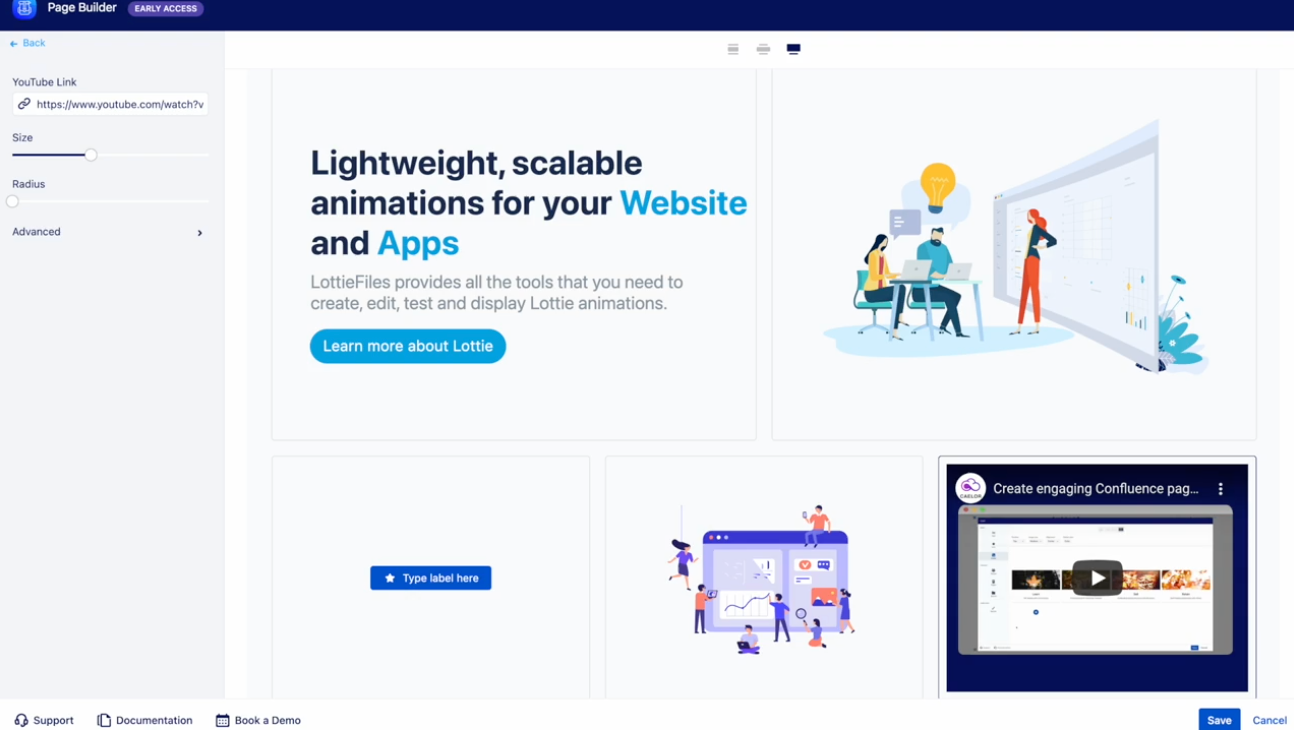This image captures the interface of a page builder website. At the top left corner, there's the text "Page Builder" rendered in white font, encased within a sleek blue bar that spans the entire width of the screen. To the left of this text, a blue logo featuring a face icon is displayed. To the right, the text "Early Access" appears next to a prominent purple button with white font.

Positioned below this bar is a back button. Directly underneath, there is a vertical menu that starts with a YouTube link, followed by another YouTube link. Beneath these links, there's an option to adjust the size, and below that is a setting labeled "Radius." Further down, an "Advanced" option is available.

Dominating the central area of the website, there is a bold statement: "Lightweight scalable animations for your website and apps." Directly below this, in a smaller font, it reads: "Lottaflies provides all the tools that you need to create, edit, test, and display Lottie animations."